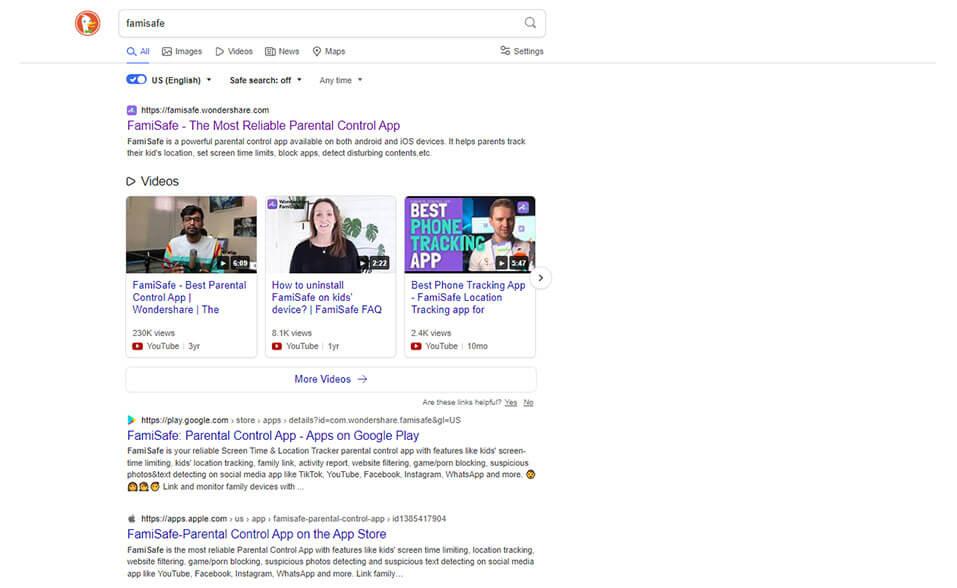The image is a horizontally rectangular screenshot of the DuckDuckGo search page. The upper left corner prominently displays the DuckDuckGo logo avatar next to the search field, which contains the query "FAMISAFE." Underneath the search field are search category options: "All," "Images," "Videos," "Docs," and "Maps." The search results are presented on the left half of the page, while the right half is blank aside from a thin gray horizontal line at the top.

The search results include three website listings followed by three video options displayed side by side. The first listed website is titled "FAMISAFE: The Most Reliable Parental Control App," highlighting its reliability. Below the website listings, we see three videos, and following these, two additional website listings: "FAMISAFE Parental Control App - Apps on Google Play" and "FAMISAFE Parental Control App on the App Store."